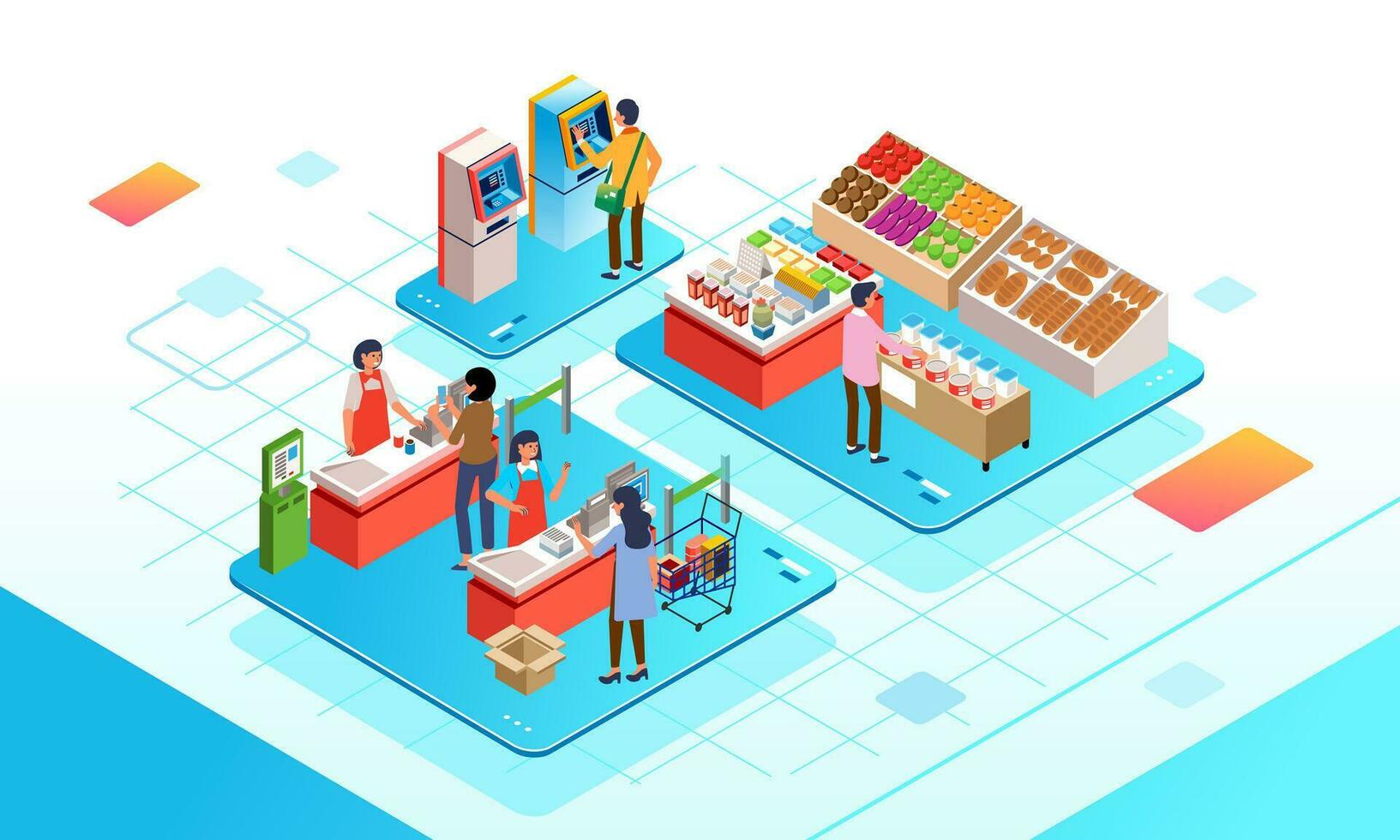The image is an isometric, vector-style cartoon illustration of a grocery store set against a large white grid background accented with light blue or teal lines. The scene is divided into floating blue rectangular panels, each representing different sections of the grocery store. The lower left panel features two checkout lanes with women in red aprons staffing the registers. One customer with a cart is being rung up at the first register, while another customer stands at the second register holding her phone. The upper left panel depicts two ATMs; a woman wearing a yellow shirt, brown pants, and a green over-the-shoulder bag is interacting with the yellow and light blue-colored ATM. The right panel displays a woman with dark hair, donning a purple or pink shirt and brown pants, examining red circular tins on a brown table amidst displays of fresh produce, baked goods, and canned items. The overall style and layout of the image evoke a futuristic, video game-like aesthetic, with the blue rectangles casting faint shadows that give them a hovering appearance above the white and teal grid floor.